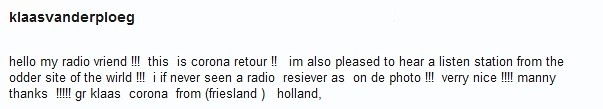The image features a plain white background with text in black font. At the top, in bold, is the name "KLAASVANDERPLOEG." Below that, in a smaller Arial font, the text reads: "Hello, my radio friend. This is Corona Retour. I am also pleased to hear a listen station from the other side of the world. I have never seen a radio receiver as in the photo. Very nice. Many thanks. GR. CLAAS. Corona from Friesland (Holland)." The message includes notable misspellings, such as "otter sight" instead of "other side," and an extended use of exclamation marks, enhancing its enthusiastic tone.